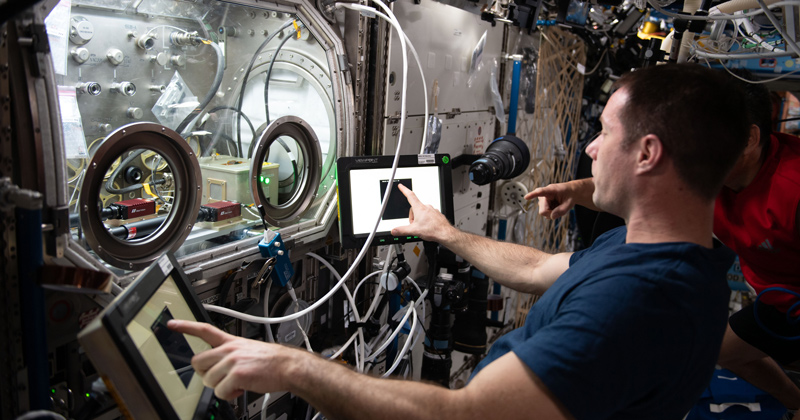The image depicts the interior of what appears to be a space station, filled with a myriad of wires, pipes, and screens. In the foreground, near the right edge of the frame, stands a man in a blue shirt with short brown hair, seen from the waist up. He faces toward the left, stretching his right arm across the bottom of the picture to touch two separate screens. Both screens have a black border with a white center, each featuring a prominent black box. He is using his index finger to interact with these screens, possibly operating some sort of device.

Directly behind him, another man, dressed in a red shirt and black shorts, partially emerges. Only his ear and a hand are visible around the first man's head, also pointing towards something. This busy, metallic environment is filled with various objects and equipment, suggesting a high-tech setting. In the left corner, there's a glass chamber with two armholes, containing numerous electrical components. The room is replete with a chaotic web of wires in various colors—blue, white, yellow, and black—amplifying the advanced scientific atmosphere of this space.